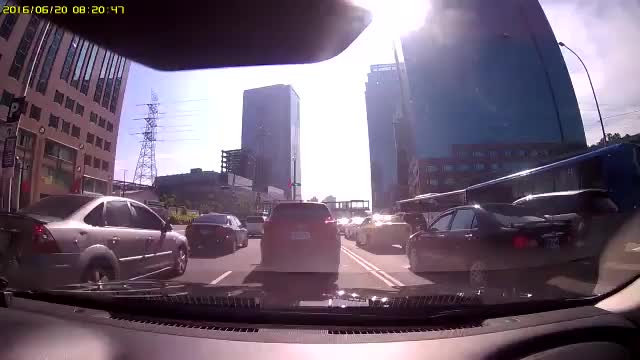A bustling cityscape unfolds through the curved windshield of a car, capturing the intricate interplay of urban elements. The multi-lane highway, clogged with dense traffic, weaves its way through a forest of towering skyscrapers. Street lights dot the scene, adding a touch of warmth amid the steel and glass edifices. A towering building dominates the background, standing sentinel over the city. The sun blazes high in the sky, casting a brilliant light that illuminates the entire scene with a radiant glow. The black front end of the car frames the bottom of the image, adding a sense of depth and motion to the composition.